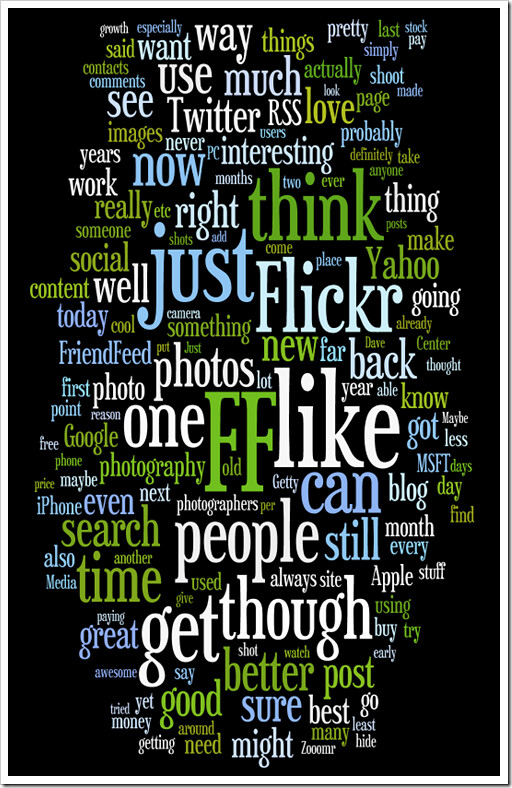This inspirational poster features a striking rectangular design in portrait mode, with a sleek, narrow white border that frames the image. The centerpiece is a stark black background adorned with a colorful array of words in vibrant shades of green, white, and blue. These words, varied in size to reflect their frequency, relate to the internet and social media. Prominent terms like "Yahoo," "FriendFeed," "Flickr," "Apple," "Google," "Photography," "Social," and "Love" stand out amongst others such as "iPhone," "Search," "Post," "Better," and "People." These words create an engaging visual mosaic, evoking themes of connectivity, innovation, and digital communication, all meticulously arranged to inspire and capture the essence of the online world.